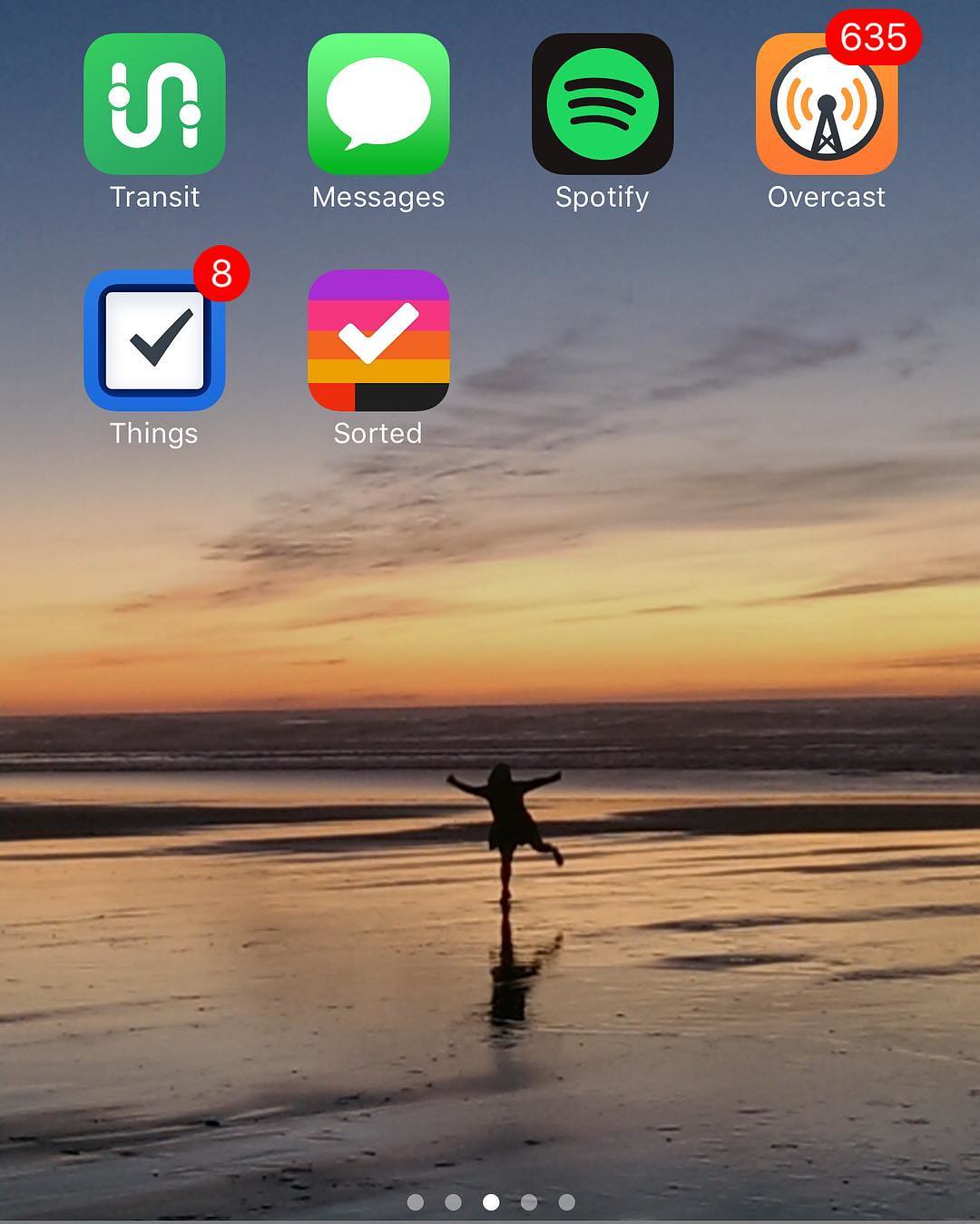This image is a potential cell phone wallpaper that could belong to either an Apple or Android device. The screen displays a series of app icons at the top. There are six app icons in total: four on the top row and two directly beneath them. 

On the top row, the first icon, labeled "Transits," features a sideways 'S' with two circles. To its right, the "Messages" app icon displays a message bubble. Next to it is the Spotify app, marked by three horizontal lines that curve upward vertically. The last app on the top row is "Overcast," represented by an antenna signal or radio tower icon.

On the row below, the "Things" app is denoted by a checkmark inside a square. Adjacent to it is the "Sorted" app, which also has a checkmark, this time white in color.

The wallpaper beneath the icons showcases the silhouette of a person, possibly a woman, rendered entirely in black. She appears to be dancing, balancing gracefully on one foot while the other foot and both arms are lifted in the air. The backdrop of the image shows a wet sandy shore with the ocean stretching out behind her. The sky above transitions from hues of purple to light orange, adding a serene and slightly whimsical atmosphere to the scene.